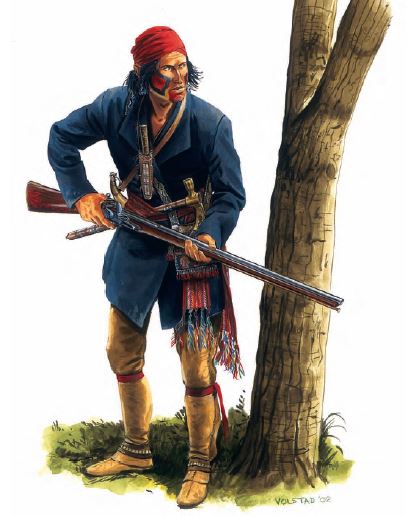This detailed illustration, possibly hand-drawn or computer-animated, features a tall Native American man, approximately six feet in height, standing next to a tree against a white background. The man has medium-length, scraggly black hair and wears war paint or face tattoos in red and blue. A red bandana adorns his head, and he is dressed in a heavy blue overcoat with lapels extending almost to his knees. His clothing ensemble includes beige pants and brown, calfskin boots decorated with red ribbons around the knees and a brown and gold anklet around the ankles.

The man appears to be in a pose suggesting stealth or anticipation, as he peeks from behind the tree, holding an old-style, single-shot rifle reminiscent of the Revolutionary or Civil War era. Supplementing his weaponry is a large knife hanging around his neck, a hammer or pickaxe attached to his belt, and a bow and arrow tucked into his waistband. A red bag with fringe also hangs from his attire. The bottom right of the image bears the signature "Volstead 02," likely indicating the artist or the year of creation. The detailed attire and weaponry suggest a readiness for combat, possibly hinting at historical conflicts involving Native Americans and the US government.